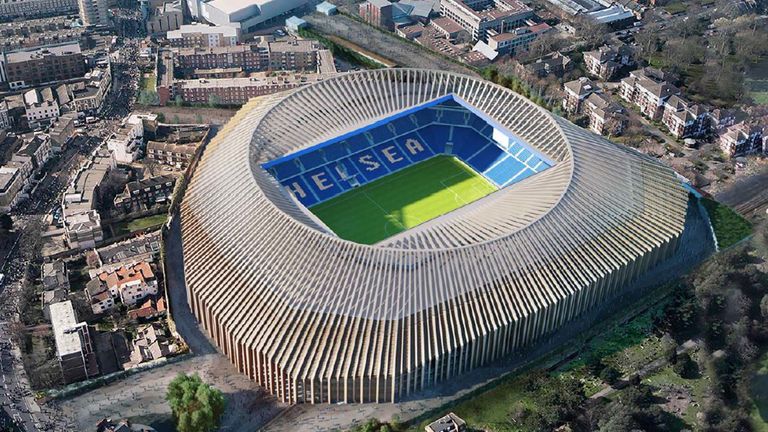This image depicts an aerial view of Chelsea's soccer stadium, an architectural marvel with a futuristic and intricate design. The stadium features a distinctive metallic exterior, with countless steel beams forming a complex polygonal structure that surrounds a square opening at the top. The beams exhibit a gradient from a silvery white at the upper sections to a tan or brown color towards the base. This sophisticated framework somewhat resembles the cage of a fan or interconnected bones.

Inside the stadium, you can clearly see the lush green soccer pitch, and the seating arrangements are predominantly blue. Stands spell out the letters "H-E-L-S-E-A" in white, forming part of the name "Chelsea," although the letter "C" is obscured from this particular aerial angle.

Surrounding the stadium is a densely packed urban area, showcasing a mix of industrial, residential, and commercial buildings. The neighborhood comprises variously sized structures, including white buildings with orange roofs and large apartment complexes. Notably, the lower-right corner of the image features a patch of green space, adorned with tall trees, adding a touch of nature to the urban landscape. Additionally, roads and possibly a railway traverse the vicinity, enhancing the depiction of this vibrant and busy area.

Overall, the photograph highlights not only the impressive stadium but also provides a glimpse into the bustling environment that encircles this iconic sports venue.